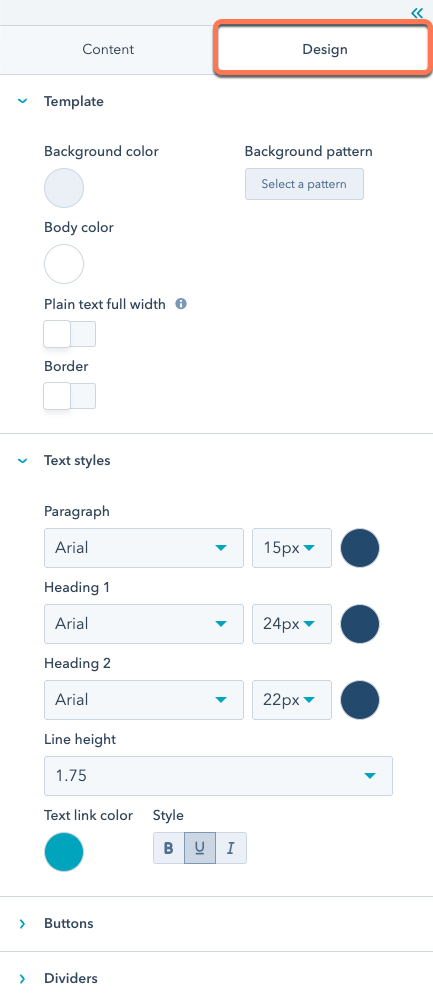The image is a screenshot captured from a mobile device, showcasing a design interface with a predominantly white background, accentuated by light blue, dark blue, and orange elements. At the top of the interface, there are two tabs: "Content" and "Design," with the "Design" tab highlighted in orange. Below the tabs, there is a section labeled "Template" accompanied by a blue drop-down arrow. 

The "Background Color" option is set to light blue, and there is an option to select a background pattern with an associated button. The "Body Color" is set to white. The interface includes options for plain text and full-width text, both of which have informational buttons circled in blue and toggles that are currently turned off.

The "Text Styles" section is displayed, featuring various text formatting options:
- For paragraph text, "Arial" is selected from a drop-down menu, with a font size of 15px and a text color of navy blue.
- For Heading 1, "Arial" is chosen from the drop-down menu, with a font size of 24px and a navy blue color.
- For Heading 2, "Arial" is selected, with a font size of 22px and a navy blue color.

Each text option is detailed with corresponding settings to ensure a cohesive design theme.